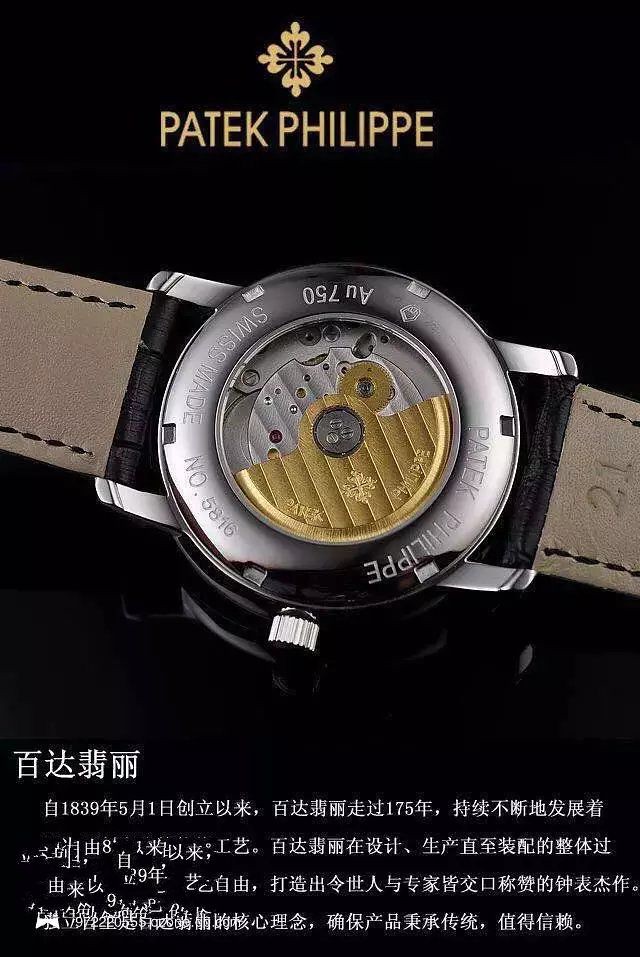The professionally crafted digital advertisement showcases a luxurious Patek Philippe watch. At the heart of the image, the watch face commands attention, adorned with a light brown leather band that extends to the mid-point on both the left and right sides. Above the watch face, a delicate flower logo accompanied by the brand’s name, "Patek Philippe," is elegantly inscribed in gold lettering. Below, Asian text adds a touch of cultural sophistication. 

The watch itself boasts a lustrous silver, or possibly stainless steel, front, with "Swiss Made" and the model number "5816AU750 Patek Philippe" clearly visible. Instead of traditional watch hands, the face features a half-circle of gold accented by intricate lettering. Beneath this, a glimpse of the watch’s inner workings is revealed, showcasing finely crafted mechanical wheels and gears set against a backdrop of textured silver metal. This detailed composition highlights the intricate craftsmanship and luxury synonymous with the Patek Philippe name.